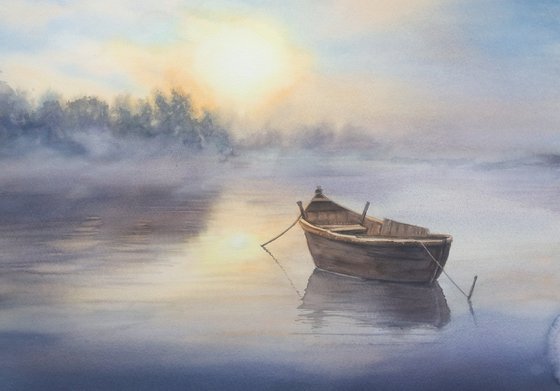This painting depicts a serene water scene, likely a river or lake, with a tranquil blue and orange tinted sky, illuminated by the setting or rising sun positioned slightly left of the upper center. Below, the sun's rays beautifully reflect off the water, creating a shimmering effect. To the right, just below the middle, a small, grayish-brown wooden boat is tied to a post protruding from the water. The boat's diagonal orientation and reflection are clearly prominent. Surrounding the water body are lush trees, bushes, and a gently sloping hill, all softly rendered with a slightly fuzzy, misty quality, enhancing the scene's quiet, almost ethereal atmosphere. The painting exudes a peaceful solitude, with no people present.